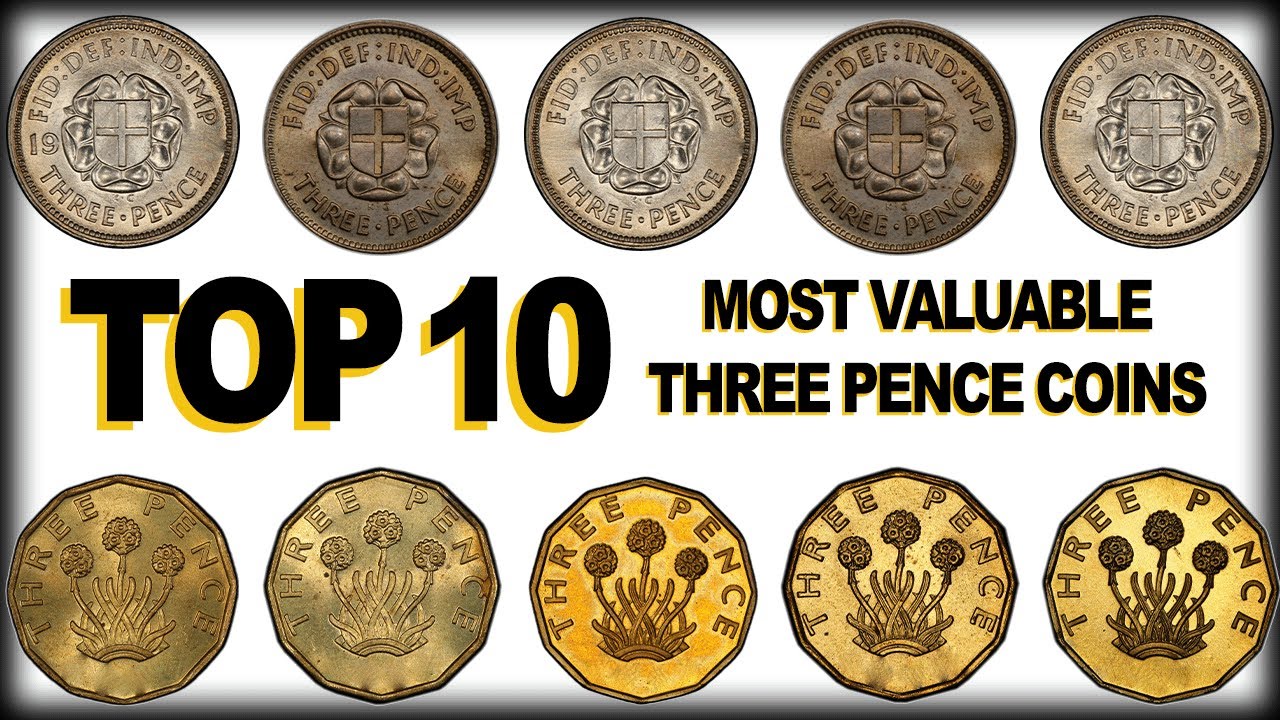This image is an illustration featuring the title "Top 10 Most Valuable Three-Pence Coins" displayed prominently in the center with black text outlined in yellow, all in capital letters. The layout is in landscape format, with two rows of coins—five at the top and five at the bottom. The top row showcases round coins in varying shades of brown to tan, with some being very dark brown and others a lighter shade of tan. The coins feature different artworks, including emblems resembling shields with several bows around them, and phrases likely in Latin, though not easily readable.

The bottom row of coins has a more yellow or gold sheen with different levels of brightness; two are dull while the one in the center is bright gold. Two coins on the bottom right also vary in brightness. These coins have slightly soft, straight edges and depict designs, including three flowers that appear to be roses, along with writing that includes the term "three pence."

Each coin provides a depiction of three-pence and varies in condition from tarnished to fairly bright, showing intricate details and historical designs from a foreign nation.